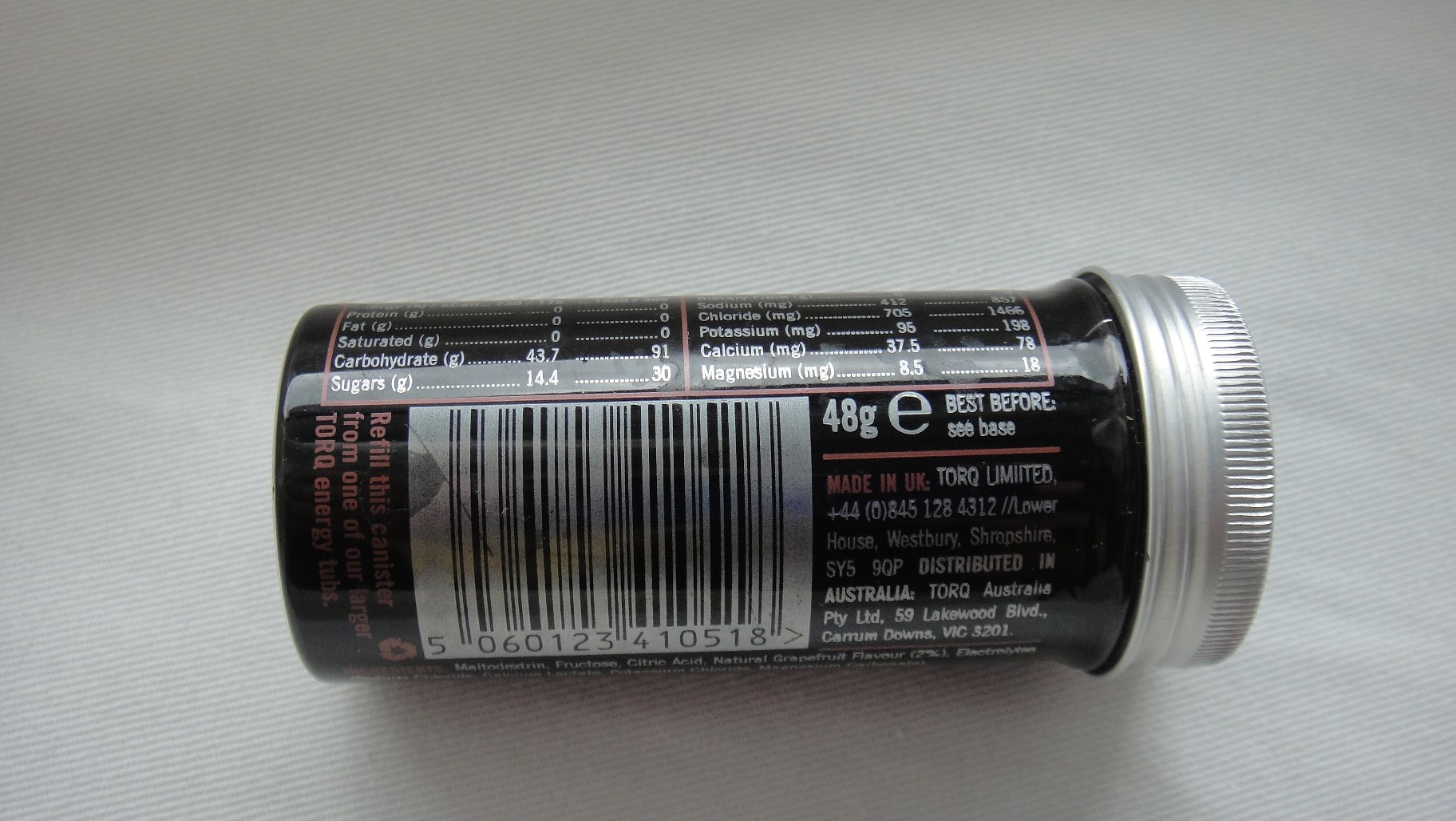This detailed color photograph captures a black cylindrical container with a textured silver screw cap, designed for easy grip with closely positioned grooves. The container lies on its side on a table, making various features visible. Prominently displayed is a large white square UPC code with black lines of varying thickness and spacing, accompanied by the numbers 5060123410518 in black. The container's label, written in white, indicates essential information such as "48 grams," "Best before: See base," and "Made in the UK by TORQ Limited," as well as instructions to "refill this container from one of our larger TORQ energy tubs." The image also reveals partial nutritional facts and additional useful details for potential users.